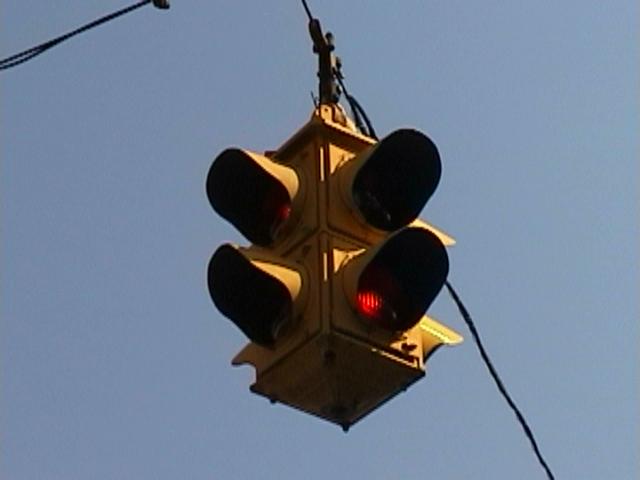In this photo, a unique four-sided traffic light hangs against a bright blue sky with no clouds. The traffic light, made of yellow metal, features two lights on each visible side, both currently showing red. We can clearly see the upper left light and the lower right light, both illuminated in red, while the other two lights are obscured in shadow. The traffic light is suspended from a black wire that extends diagonally from the bottom right to the upper left of the image. The overall scene is devoid of any text or additional street elements, focusing solely on this distinctive traffic signal.